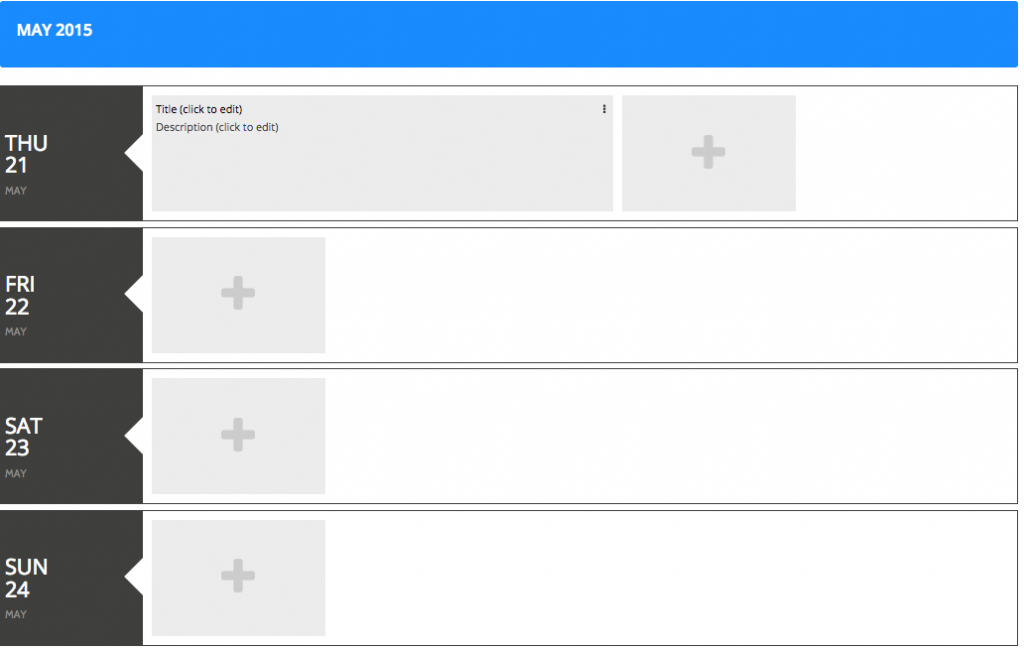The image is a screenshot of a digital calendar or date-related interface from May 2015. The top bar of the interface is blue, and on the top left corner, white text displays "May 2015". Below this header, there are four rows, each representing different days of the month.

1. **Thursday, May 21, 2015**: The first row features a gray box on the left labeled "Thursday, 21st May". To the right, there is a clickable area labeled "Title to edit" followed by a description field labeled "Click to edit." On the far right, there is a plus icon indicating an option to upload or add content.

2. **Friday, May 22, 2015**: The second row mirrors the format of the first, with a gray box on the left marked "Friday, 22nd May". Adjacent to the gray box is empty white space, indicating that no content has been added. Again, a plus icon is present.

3. **Saturday, May 23, 2015**: For the third row, "Saturday, 23rd May" is displayed in a gray box on the left. Beside this, there is a lighter gray box containing a plus sign, and a significant amount of empty white space to the right.

4. **Sunday, May 24, 2015**: The bottom row shows "Sunday, 24th May" within a dark gray box. Similar to the previous rows, there is an adjacent lighter gray box with a plus sign, followed by ample empty white space.

All the days listed contain no additional content, suggesting that the calendar entries have yet to be filled out.